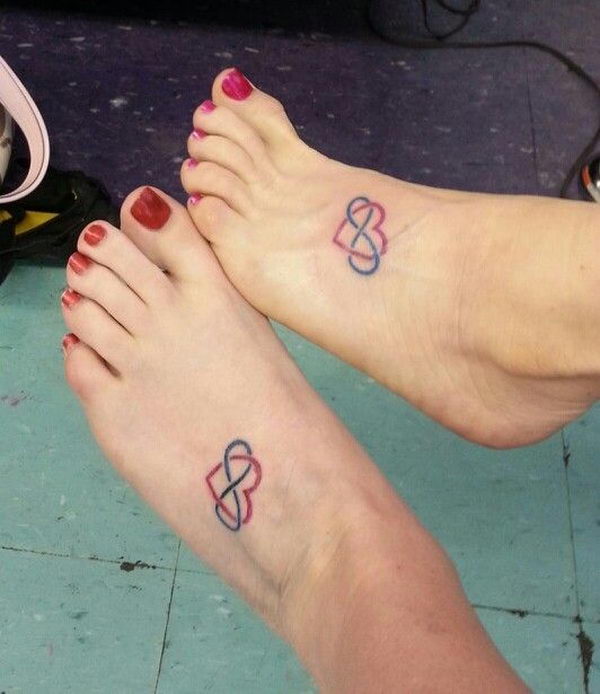In the photo titled "Token Inside," two feet from different people are featured prominently. These are left and right feet, one appearing larger than the other. Both feet are adorned with dark red nail polish and have matching tattoos, consisting of a red heart intersected by a dark infinity ring. The feet, both fair-skinned, are in close proximity, with the smaller foot resting against the larger. The scene is set against a backdrop of white and darker gray vinyl tiles.